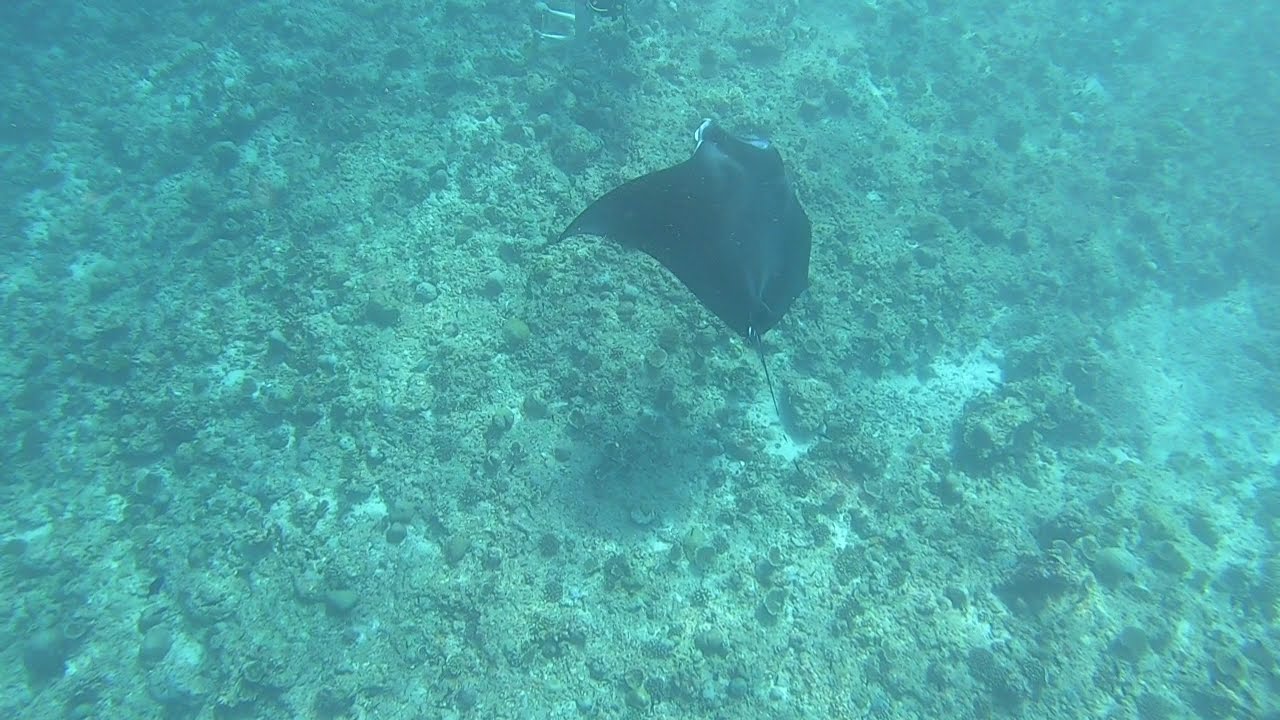The image, taken underwater, reveals a slightly unclear, hazy scene with greenish-blue water. The central focus is a majestic manta ray, gliding gracefully above a rocky ocean floor. The manta ray, predominantly black with some white on its underside, displays its long tail and distinct fins. Beneath it, its shadow is cast clearly on the bottom surface. The ocean floor is strewn with rocks, flat coral, and debris, giving it a rugged appearance. In the top portion of the image, parts of a person's legs are visible, suggesting a diver or swimmer nearby, appearing much smaller in scale compared to the imposing manta ray.